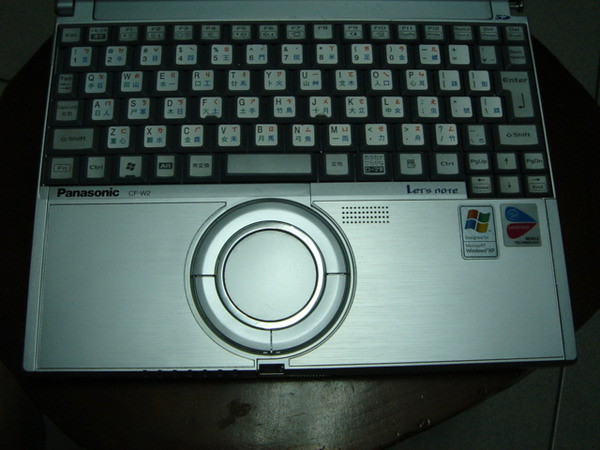The image depicts an overhead view of an older Panasonic CF-W2 laptop, seated on a wooden table with a tiled floor partially visible around it. The laptop is notable for its unique circular touchpad, which is surrounded by one large button covering the upper half and two smaller buttons for left and right clicks on the lower half. The laptop is primarily metallic gray with a clean, well-preserved keyboard that includes both English letters and Japanese characters in green, blue, and red. On the bottom right corner of the laptop, there are two stickers: one indicating it runs Windows XP and another with a blue and red teardrop shape. The edges of the keyboard are silver, while the keys themselves are a mix of white and gray, with functional keys like "shift," "ctrl," and "fn." The Panasonic branding is clearly visible on the left side of the keyboard area, emphasizing its Japanese origin. The entire keyboard is in view, though the screen is not, giving a detailed look at the distinctive design and multilingual capability of this vintage laptop.